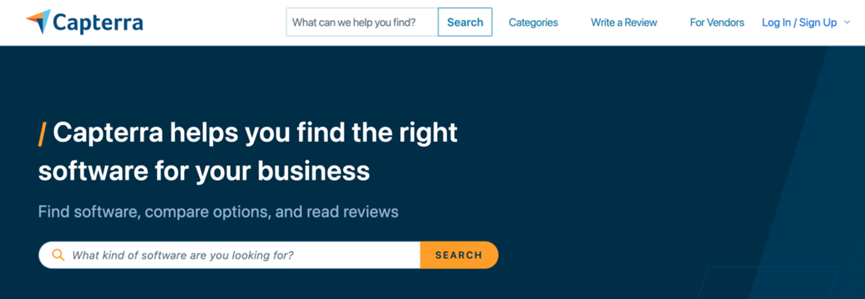The image displays the homepage of the Captura website against a clean, white background. At the top-left corner, there is a logo resembling an arrowhead or a send icon with colors orange, blue, and dark blue. To the right of the logo, "CAPTERRA" is prominently displayed in dark blue letters, followed by a blank white space. Further right, there's a search bar with the text "What can we help you find?" inside, and the word "Search" in blue letters, outlined in blue.

Continuing from left to right, there are navigation options including "Categories," "Write a Review," "For Vendors," and "Log In/Sign Up", all written in blue letters. Below this top navigation, a dark blue rectangular banner spans the width of the page, with its right side and bottom right corner shaded lighter blue. An orange forward slash appears at the left edge of the banner, followed by the phrase "Capterra helps you find the right software for your business" in white letters. Beneath this, a secondary message in blue letters reads, "Find software, compare options, and read reviews."

Positioned towards the left side of this dark blue rectangle is a white search bar featuring an orange magnifying glass icon. Inside the search bar, the prompt "What kind of software are you looking for?" is displayed in blue letters. To the right of this search bar, the word "Search" is written in bold black letters on an orange background.